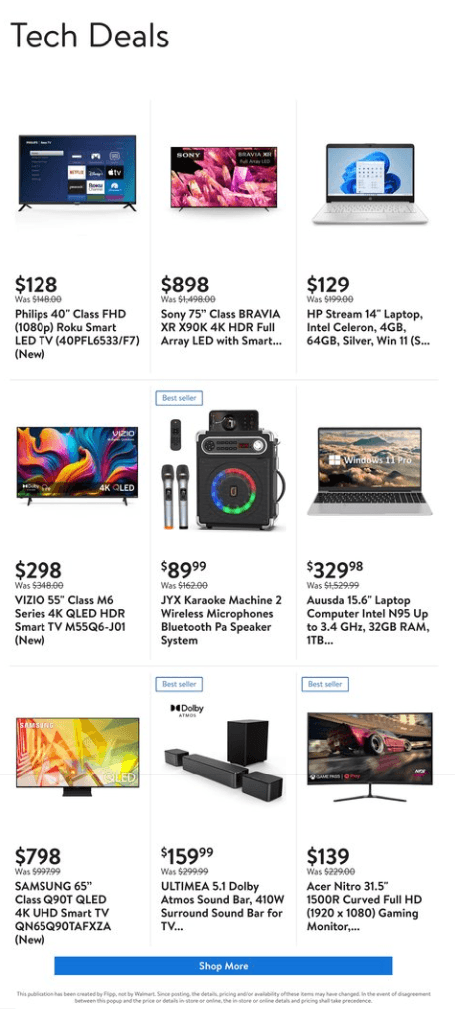**Tech Deals Showcase**

Set against a clean white background, the words "Tech Deals" are prominently featured in black at the top left corner. The display presents nine different deals arranged in three columns, each featuring high-tech products with significant discounts. Below is a detailed breakdown of the deals:

**Column 1:**
1. **Philips 40-inch Class FHD 1080p Roku Smart LED TV**  
   - Price: $128 (previously $148, now crossed off)
   - Tag: **New**
   - Excitement Note: "How could it be that cheap?"
   - Image: Shows a sleek flat-screen TV.

2. **Sony 75-inch Class Bravia XR X90K FK HDR Full Array LED Smart TV**  
   - Price: $898 (previously $1498)
   - Image: Depicts a large high-definition flat-screen TV.

3. **HP Stream 14-inch Laptop**  
   - Price: $129 (previously $199)
   - Specs: Intel Celeron, 4GB RAM, 64GB storage, Silver finish, Windows 11
   - Image: Displays a sleek silver laptop.

**Column 2:**
1. **Vizio 55-inch Class M6 Series 4K QLED HDR Smart TV**  
   - Price: $298 (previously $348)
   - Tag: **New**
   - Image: Shows a vibrant, high-resolution TV screen.

2. **JYK Karaoke Machine**  
   - Price: $89.99 (previously $162)
   - Features: Includes two wireless microphones and a blue PA speaker system
   - Tag: **Bestseller** on a blue banner
   - Image: Highlights the array with two microphones.

3. **AUUSDA 15.6-inch Laptop Computer**  
   - Price: $329.98 (previously $1529.99)
   - Specs: Intel N95 up to 3.4 GHz, 32GB RAM, 1TB storage, Windows 11 Pro
   - Image: Displays a high-performance laptop.

**Column 3:**
1. **Samsung 65-inch Class Q90T QLED 4K UHD Smart TV**  
   - Price: $798 (previously $997.99)
   - Tag: **New**
   - Image: Features a stunning flat-screen TV.

2. **Ultimate 5.1 Dolby Atmos Soundbar**  
   - Price: $159.99 (previously $299.99)
   - Specs: 410W surround sound for TV
   - Tag: **Bestseller** on a blue banner
   - Image: Shows the complete soundbar system setup.

3. **Acer Nitro 31.5-inch 1500R Curved Full HD Gaming Monitor**  
   - Price: $139 (previously $229)
   - Tag: **Bestseller** with a blue ribbon
   - Image: Illustrates the immersive curved gaming monitor.
   - Note: There's a **Shop More** button in white at the bottom.

A final note at the bottom of the publication reads: "This publication has been created by Slip, not by Walmart," with additional blurry sentences following.

---

This detailed description provides a clear and comprehensive picture of the tech deals and their standout features.